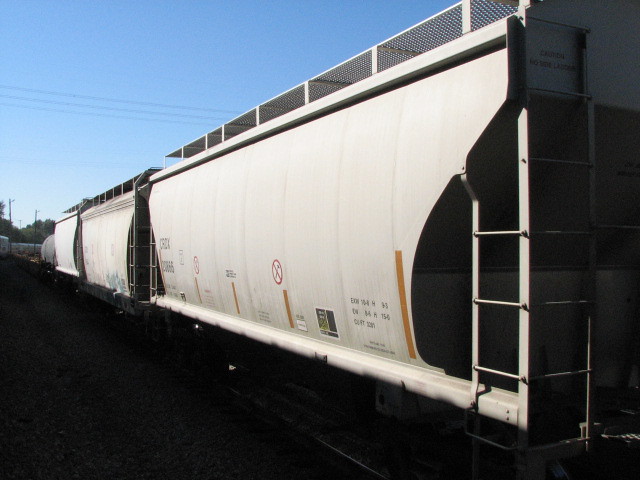This color photograph captures an extensive lineup of large white freight containers, slightly rectangular with curved sides, positioned along a black paved road. Each container features a small ladder on one side and black writing, which is too small to decipher. The containers are equipped with a top rectangular piece, supported by square welded sections along metal grating, facilitating inspection access. All three containers share this setup, with the container in the middle displaying blue graffiti on its bottom part. In the background, beyond these containers, another large cylindrical container, light brown in color, is visible. There are additional distant containers and buildings, but they appear small and blurry due to the distance. The scene is set during a sunny day with a clear blue sky, and a line of dark green trees can be seen towards the center left. The photograph also reveals three telephone lines stretching across the left of center, contributing to the landscape's depth. Additionally, a partially visible red circle with an item crossed out can be spotted on one container, though its details remain unclear. The freight cars appear to extend infinitely into the distance, slightly veering to the right and continuing out of view, emphasizing the photograph's vast landscape perspective.